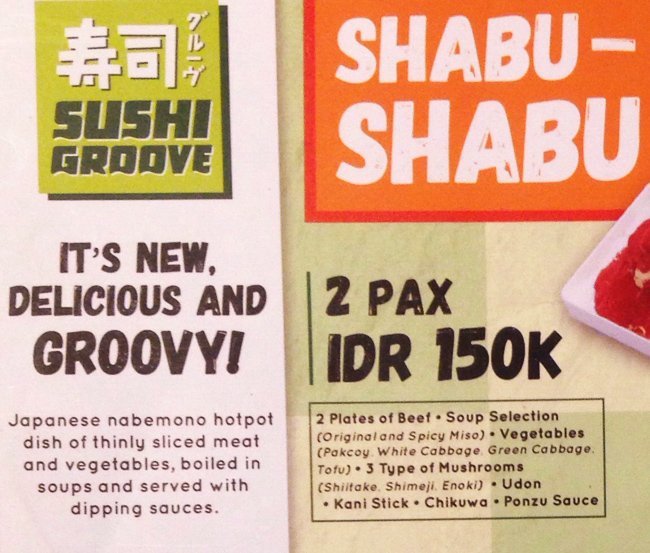This image shows a detailed, slightly worn and grainy menu from a sushi restaurant, laid flat and divided into two sections. On the left side, there's a green box at the top with white text that reads "Sushi Groove." Below, on a light pink background, it promotes this new and delicious Japanese Nabemono hot pot dish of thinly sliced meat and vegetables, boiled in soups and served with dipping sauces. On the right side, against a tan background, there's an orange box at the top with white text that says "Shabu Shabu." Below that, in black text, it offers "Two Packs" for IDR 150K, detailing that this includes two plates of beef, a selection of soups (original and spicy miso), vegetables (pak choi, white cabbage, green cabbage), tofu, three types of mushrooms (shiitake, shimeji, enoki), udon, kani stick, chikuwa, and ponzu sauce.